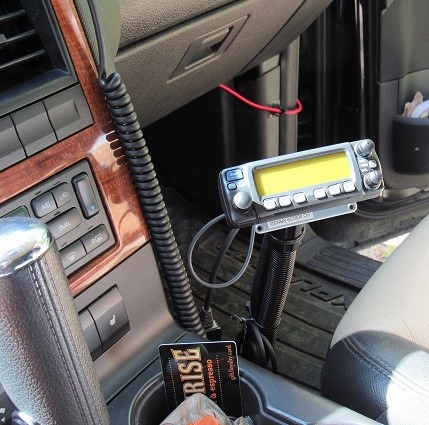The image displays an interior photograph of an old car, presumably a 1990s taxi cab, evidenced by a small mount on the passenger side. The focus is on the center console, featuring a faux mahogany panel, black plastic buttons with white symbols, such as an AC button and a defroster symbol. The console also shows some exposed wiring, perhaps from a theft attempt. The console aesthetic reflects an undigitized era with multiple manual buttons and air vents with horizontal plastic blades.

In the cup holder, there is a likely coffee shop gift card that prominently reads "RISE" in uppercase letters and "espresso" in lowercase. The glove compartment is partially visible with a distinctive square-shaped opener beside an open passenger door showing a black plastic storage pocket. The seats are black with a white seating area.

Additional features include a yellow digital meter, indicative of older technology, and wires protruding throughout suggesting some disarray. The overall black and gray interior supports the vehicle's vintage appearance.